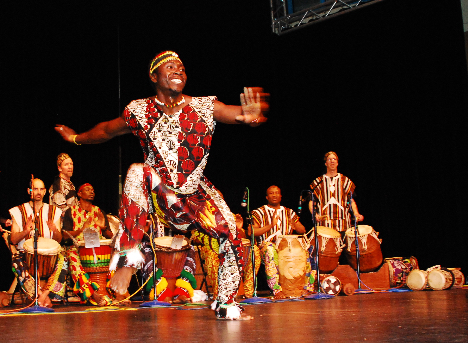This indoor photograph captures a vibrant performance, centering on a male dancer with brown skin, clad in traditional African attire that includes a colorful head wrap adorned with yellows, greens, gold, and red. His outfit features a striking red, black, and white patterned design with long pants. The dancer is in mid-motion, creating a blurred effect as he enthusiastically moves with one arm extended forward and the other back, while his beaming smile radiates joy and energy. His left knee is bent and planted firmly on the stage, which is dark and shiny, complementing the dynamic scene. Behind him, a row of musicians, some of whom are white, are similarly attired in colorful African garbs, predominantly in shades of red, yellow, brown, and black. These musicians are playing large drums, possibly bongos, and are equipped with black microphones, indicating a professional performance setup. The backdrop consists of black curtains with visible metal supports near the top right, framing this captivating display of cultural expression.